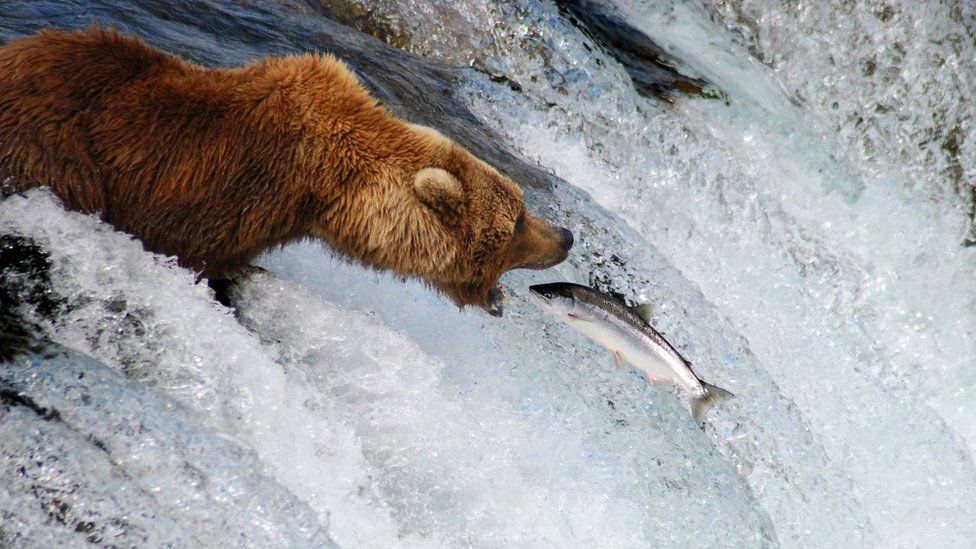In this breathtaking nature photograph, a reddish-brown grizzly bear stands poised among the frigid, rushing waters of a steely blue waterfall. The waterfall, cascading downward with white cresting foam, provides a dramatic backdrop. On the top left of the frame, the bear stands with an arching back, its lighter brown ears perked forward. The bear's head, darker in contrast, faces to the right with jaws wide open, revealing three small white teeth in the lower jaw and a dark black nose. Positioned face-to-face with the bear, a sleek silver salmon, identifiable by its black pointed head and prominent fins, jumps upstream seemingly directly into the bear’s gaping mouth. The bear is strategically situated within the icy, foamy rapids, ready to catch its meal in this striking moment captured in nature.